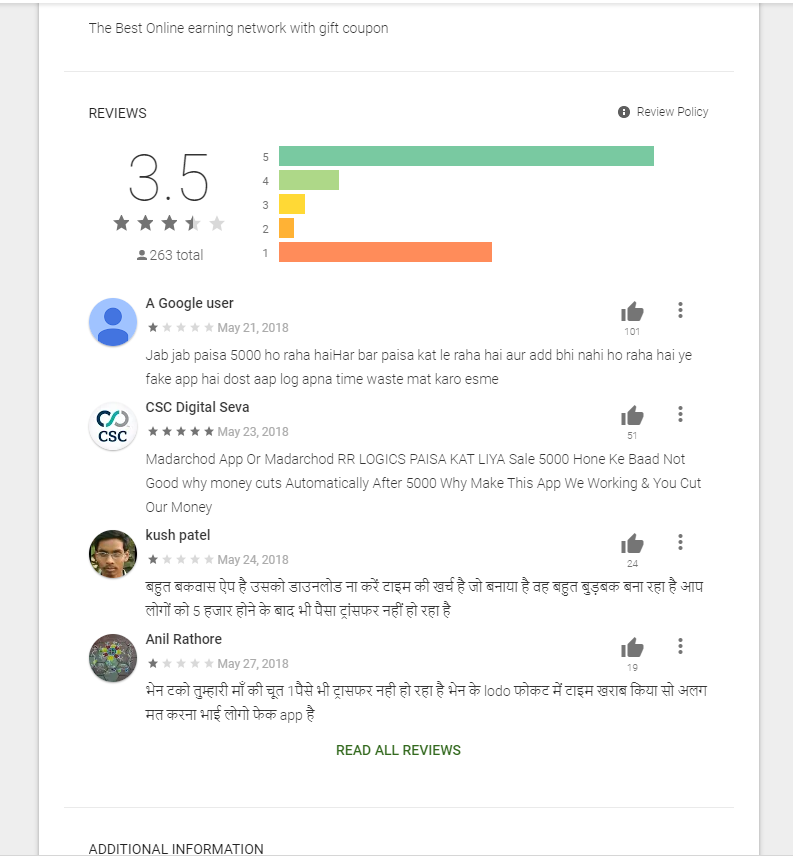This image showcases a Google Reviews page with detailed user feedback and a star rating summary. On the left, the overall rating is 3.5 stars, derived from the input of 263 users. To the right, a horizontal bar graph is displayed, labeled from 5 stars at the top down to 1 star at the bottom. The 5-star rating bar, colored green, is the most prominent, indicating a significant proportion of positive feedback. Conversely, the second most prominent bar is the 1-star rating, shown in orange, followed by the 4-star rating, which is depicted as a light green bar.

Below the graph are four reviews in a foreign language from different users. The top review is by an anonymous Google User, posted on May 21, 2018, earning 101 likes but giving a 1-star rating. Next, CSC Digital Seva posted a 5-star review on May 23, 2018, receiving 51 likes. The third review is by Kash Patel, posted on May 24, 2018, also giving a 1-star rating with 24 likes. Finally, Anil Ratore's review, dated May 27, 2018, gave 1 star and garnered 19 likes. 

At the bottom center of the page, there is green text stating "Read all reviews," encouraging users to delve further into the feedback. The page itself has a white background. Positioned at the top right, adjacent to the bar graph, is an information icon labeled "Review policy."